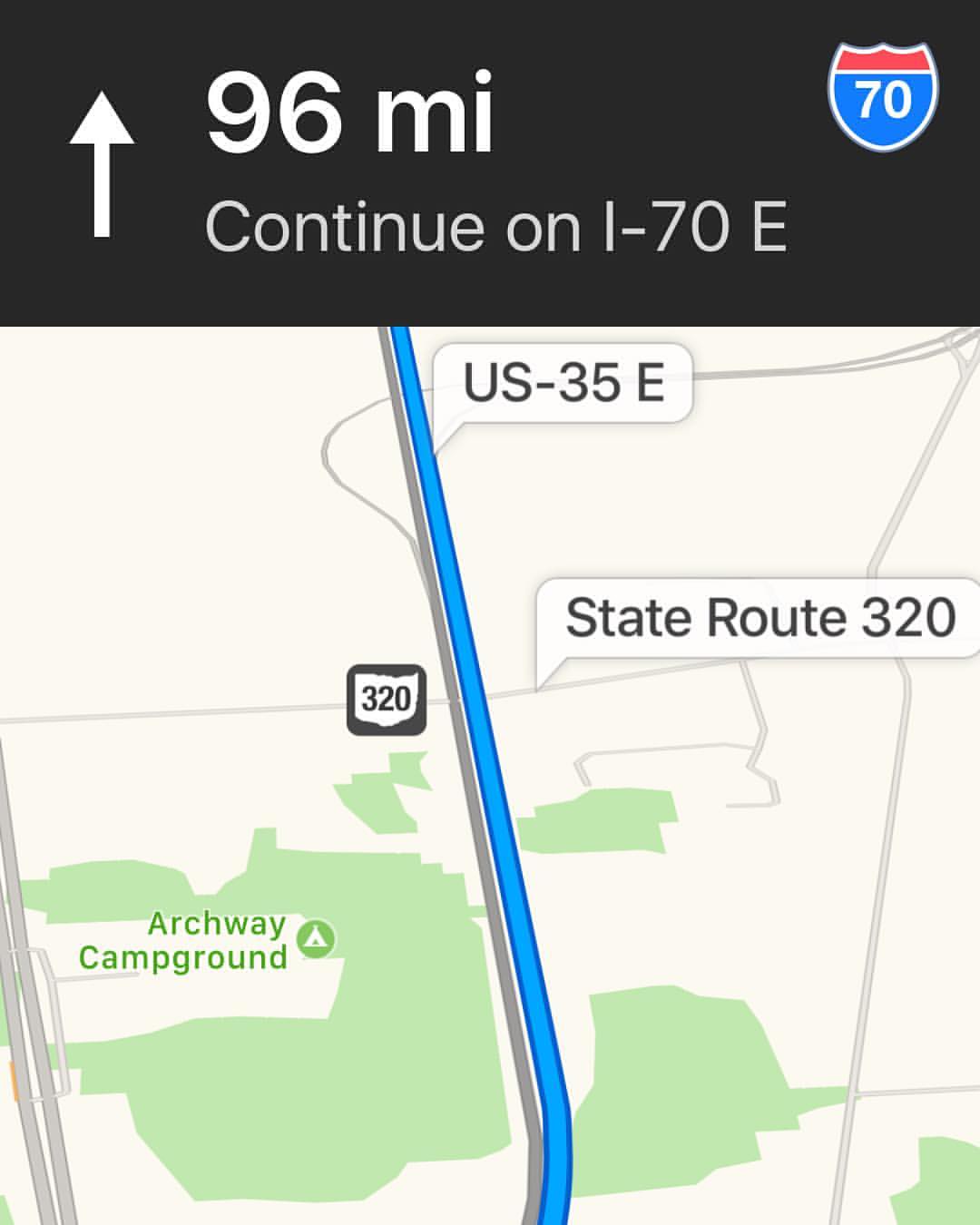This image showcases a map, likely sourced from a GPS system, highlighting various geographical and infrastructural details. Prominently, a blue line, denoted as US 35E, runs vertically from the bottom to the top of the image, bisecting the map with notable straightness. Green areas, representing parks or natural reserves, are scattered across the map, adding visual contrast. Gray straight lines on both the left and right sides indicate additional roads, with one vertical gray line intersecting the blue line, specifically marked as State Route 320. A notable landmark, Archway Campground, is labeled on the left side near one of the green areas. Dominating the top of the image, a black rectangle contains a white forward-pointing arrow on the left, accompanied by the text "96MI" next to it. Below this, instructions read "continue on I-70E," supported by an icon featuring a blue field with a red banner and the number 70 inside, guiding the viewer on their journey.